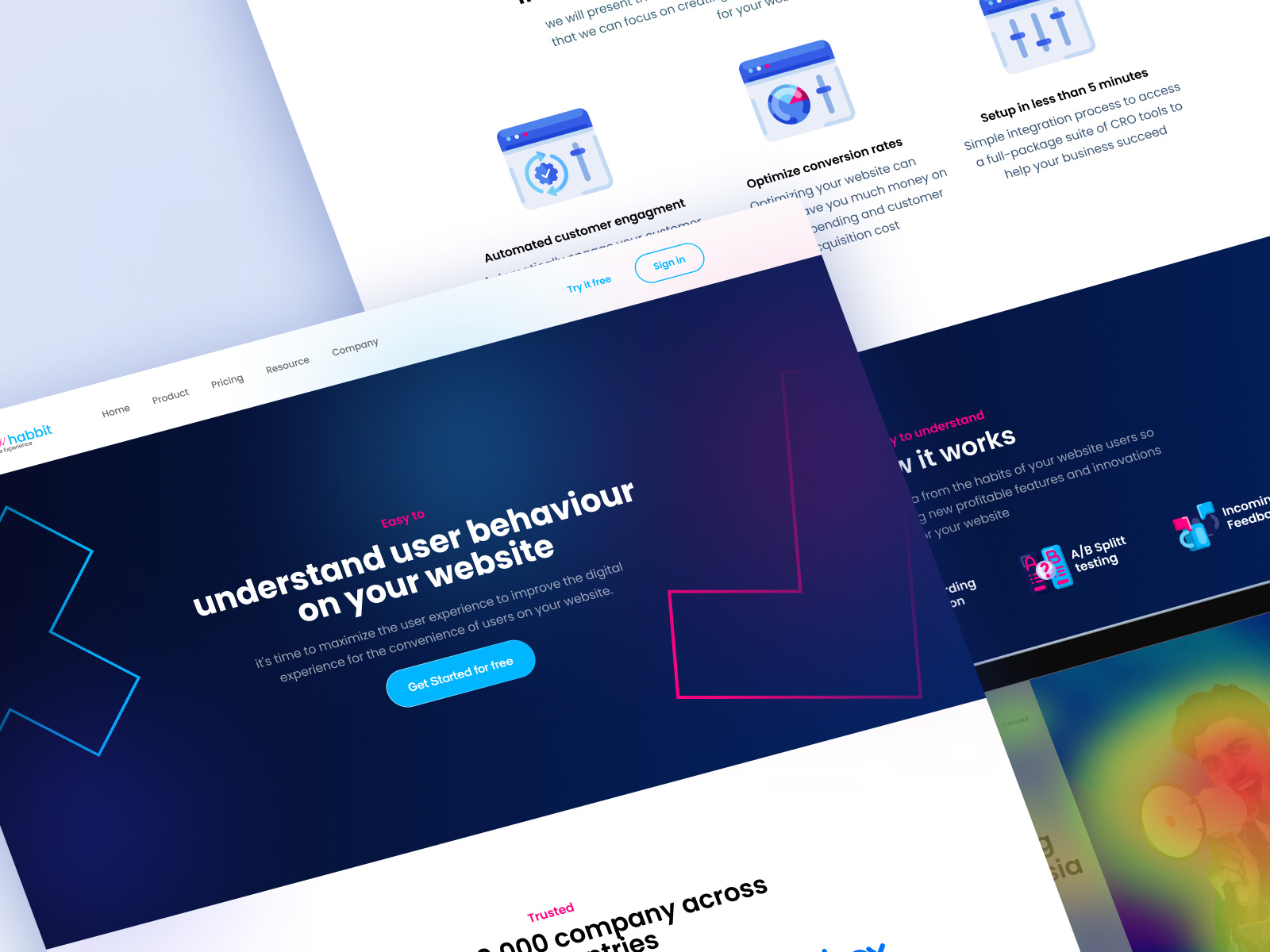The image displays a composite view of various screen captures. On the left side of the background, there is a grey panel containing several menus. To the right of this panel, a series of bar charts and interactive levers are visible, which likely represent controls for different functionalities. Specifically, there are headings indicating features such as "Automated Customer Engagement," "Optimized Conversion Rates," and "Setup in Less Than Five Minutes."

Overlaid on this background is a screenshot of a webpage from a site identified by blue lettering in the top left corner as "Habit." This page contains a horizontal navigation menu with options like "Home," "Product," "Pricing," and a partially obscured item, followed by "Company." Additionally, there are prominent blue links for "Try It Now" and a "Sign In" button.

Below the navigation bar, the webpage includes a dark blue splash screen adorned with two abstract shapes on either side. Central to this splash screen is white text that reads, "Understand User Behavior on Your Website." Beneath this text is a blue button labeled "Get Started for Free."